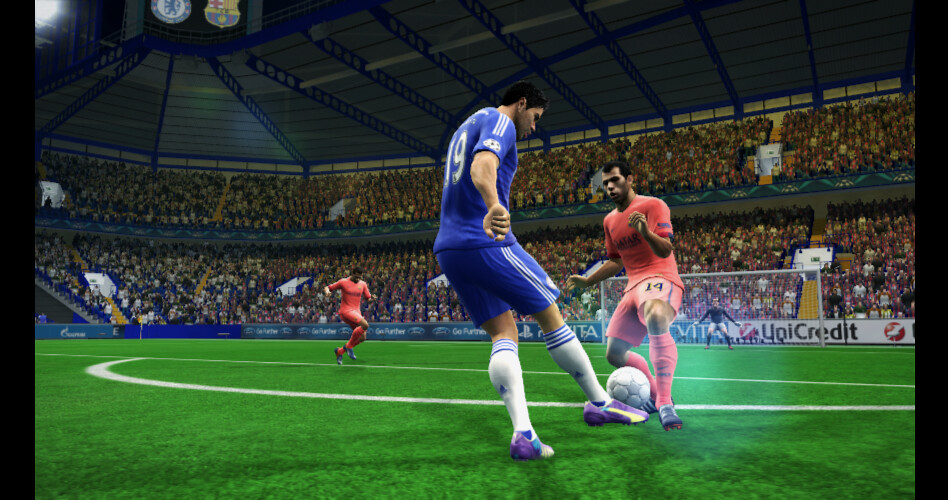The image depicts a detailed and lifelike scene from a video game of an indoor soccer match in a large, vibrant stadium filled with cheering fans. The field features vividly green grass with white lines and markings. Overhead, the stadium's blue and silver roof is adorned with prominent lights, illuminating the energetic scene below. In the foreground, a goalie stands alert in front of a wide net, donned in a black shirt, gray shorts, long black socks, and white gloves. A player wearing a blue jersey with the number 19, white and blue socks, and purple and white cleats is captured mid-action, seemingly having just kicked the white and gray soccer ball. Opposing him is a player clad entirely in a vibrant orange-red uniform with the number 14 displayed in black, and tall socks, also poised to make a move. The excitement of the game is palpable with other players visible on the field and the crowd's energy contributing to the lively ambiance of this immersive video game moment.